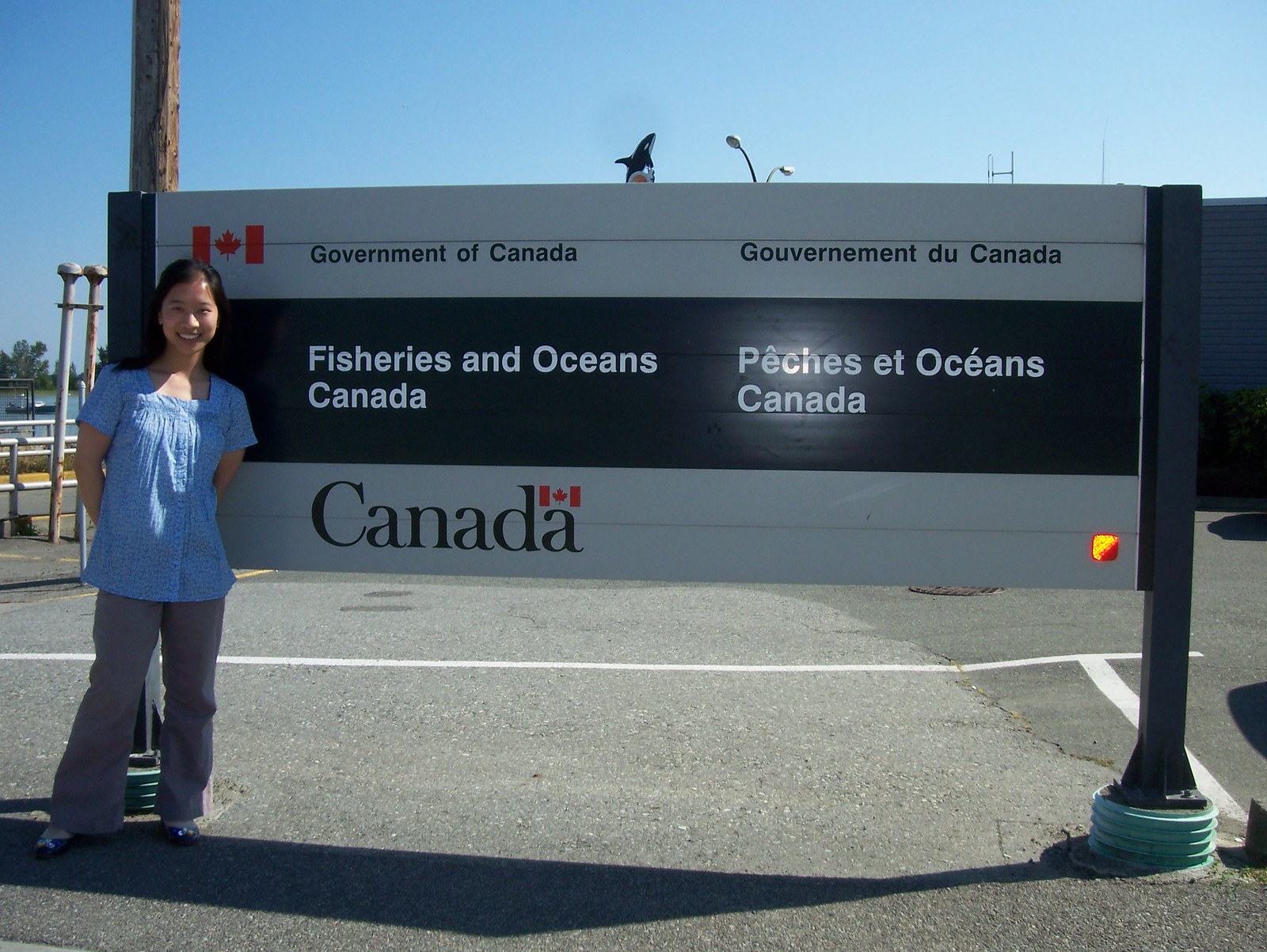In this outdoor photograph taken in a presumed parking lot near a waterfront, an Asian woman, possibly in her late teens or early 20s, poses to the left of a large Government of Canada sign. She sports long, black hair and a stylish outfit consisting of a blue and white blouse, grey bell-bottom pants, and dark blue slip-on shoes. The prominent sign, which occupies most of the center of the image, features the Canadian flag in the top left corner and bears the bilingual text: "Government of Canada" and "Fisheries and Oceans Canada." At the bottom, "Canada" is written with another small Canadian flag above the "A." The setting is bright with a clear, sunny blue sky, and the background includes a wooden telephone post, a pair of streetlights, and a distant view of a lake.